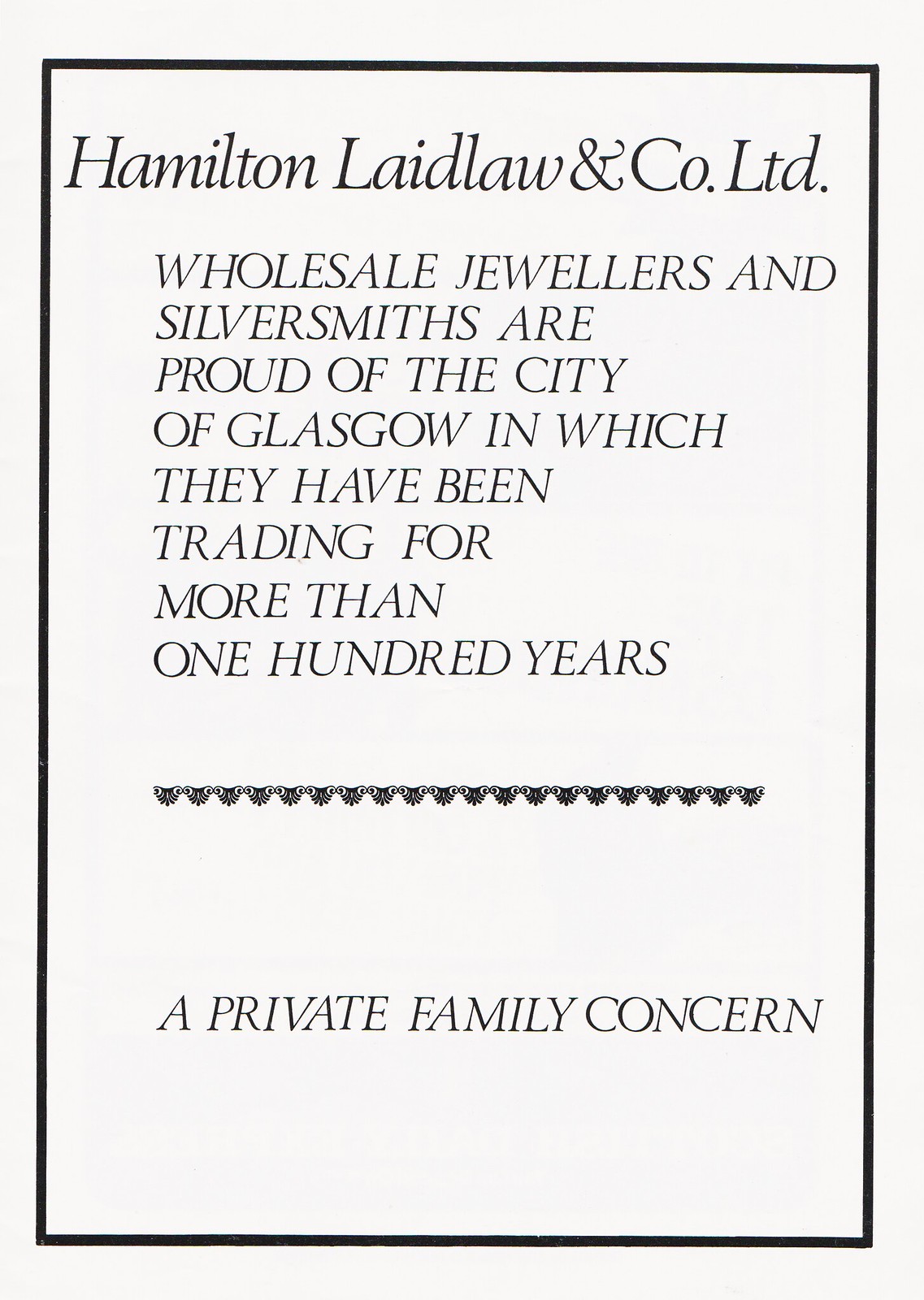The image showcases a vertically aligned rectangular advertisement or cover page set against a light gray background. It features a prominent black border surrounding the main content, which is presented on a blank white page. At the top, in left-aligned black text, it reads "Hamilton, Laidlaw, and Co. LTD." Below this, centered text proudly states, "Wholesale Jewelers and Silversmiths are proud of the City of Glasgow, in which they have been trading for more than 100 years." A decorative, lacy-looking black line divides the text, and at the bottom, also centered, it concludes with "A Private Family Concern." There are 20 small icons, resembling ox heads, arranged horizontally across the lower part of the page.